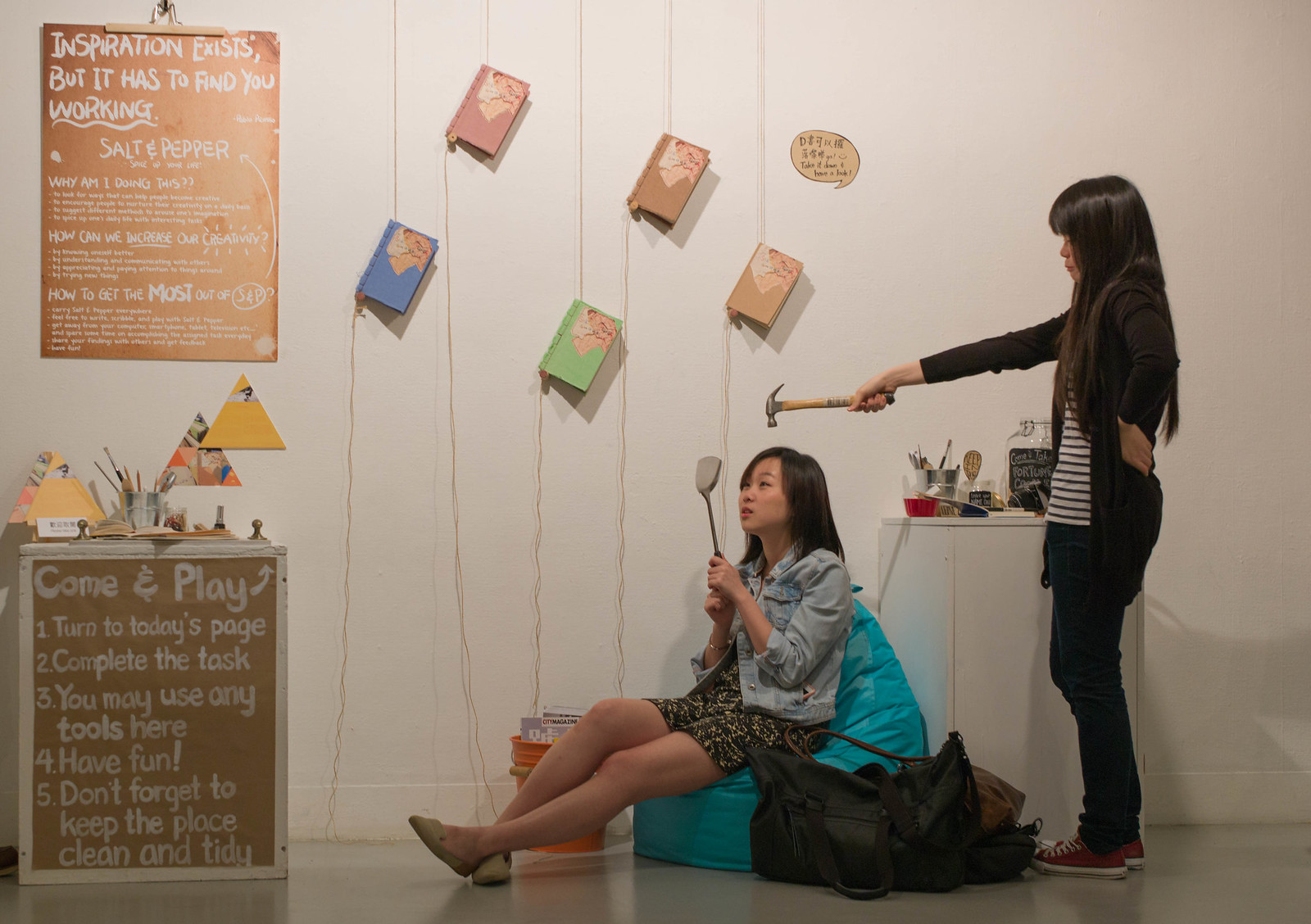The photo depicts two girls posing in a minimally decorated room. The central focus is on the girl seated on a small bean bag or blue futon, who holds up a spatula-shaped mirror to her face and gazes at it hypnotically. Standing behind her, the second girl holds a hammer in her right hand, poised as if to strike the seated girl’s head. The room features five books hanging from strings on the wall, adding whimsical décor. On the left side, two green boards display motivational texts, with one board stating, "Inspiration exists, but it has to find you working," and the other instructing, "Come and play. Turn to today's page. Complete the task. You may use any tools here. Have fun. Don't forget to keep the place clean and tidy." There are also bags placed on the floor next to the girls, and a table or similar furniture item is visible in the bottom left corner. The photo captures a quirky and staged scene, set in what appears to be an activity or creativity room.